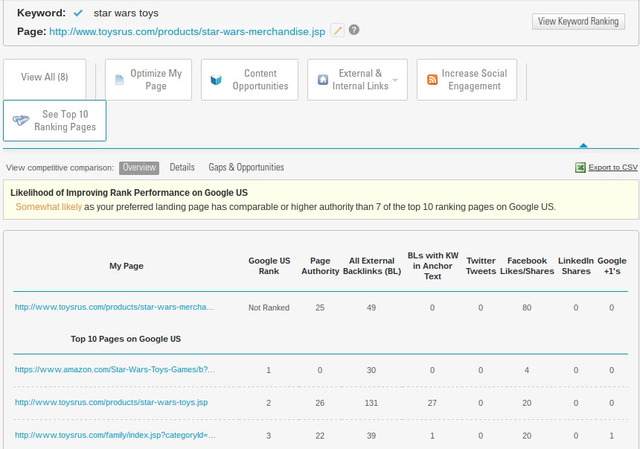The image depicts a webpage focused on keyword rankings, specifically for "Star War Toys". The top of the webpage features a light blue background with a black banner across the top left corner. Within this banner, the header "Keyword" is displayed in black text, followed by a blue arrow, and then the term "Star War Toys" in black text. To the right, there is a light-colored banner that reads "View Keyword Ranking" in dark letters.

Below the banner, the word "Page" is prominently displayed in black, accompanied by a light blue web address. Adjacent to this is a small pencil icon indicating the option to edit, as well as a circular question mark symbol.

The main section of the webpage contains five distinct white rectangles, each with blue text. The first box on the left reads "View All 8" (with the number 8 in parentheses). Moving from left to right, each subsequent box contains different information. Beneath these rectangles, there is a larger box labeled "See Top 10 Ranking Pages".

Further down, the page discusses the likelihood of improving rank performance on Google U.S. Below this section, there is a list displaying different webpages, each highlighted in bright blue text. These entries are likely related to Star Wars toys, with columns indicating various metrics such as "Rank U.S.", "Rank", and "Page Authority" alongside respective numerical data.

Towards the bottom, additional webpages with similar formatting and bright blue highlights are presented, suggesting a detailed ranking analysis layout.